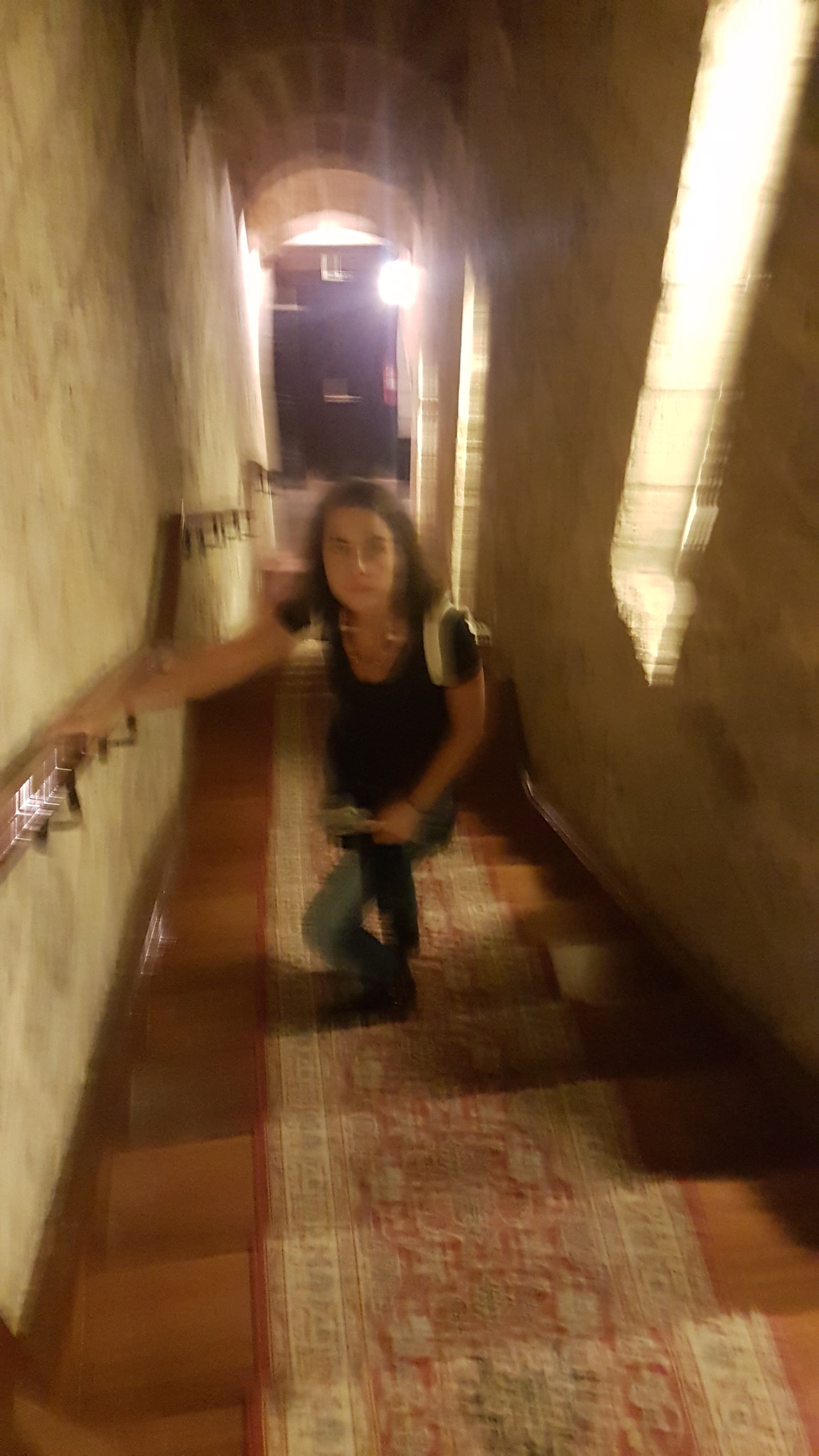This photograph features a young woman standing midway on a staircase, facing the camera with a stoic expression. Her shoulder-length brown hair frames her face, which is devoid of bangs. She grasps the stair railing with her right hand, poised on the carpeted steps. The carpet runner, extending the full length of the wooden staircase, provides a striking contrast against the rich wood beneath. To her left, a window lets in a soft light, illuminating her from the side, while to her right, a beige wall forms the backdrop against which she holds the railing. The overall image is quite blurry, rendering details indistinct and ethereal.